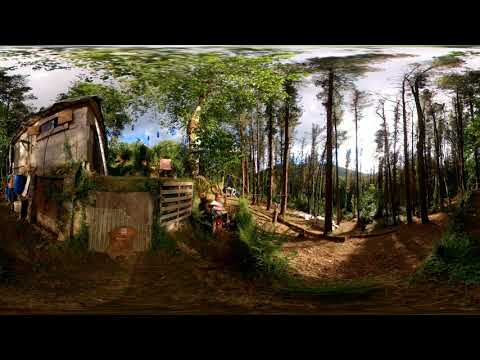This image captures a serene outdoor scene, depicting a forest area with tall, straight trees, some abundant with leaves and others almost bare, their foliage scattered on the ground below. The ground itself is a mix of light brown and reddish soil, interspersed with sticks, fallen leaves, and patches of green grass. The sky above is a blend of blue and white, indicating daytime with sunlight filtering through the trees and dappling the earth below. In the background, an old, run-down house made of wood panels and pallets stands prominently. It is a two-level shack, weathered and worn, adding an element of rustic charm. Not far from the dwelling, a pallet serves as a makeshift fence, and a wooden chair is positioned outside. A man is seated there, seemingly enjoying the tranquil view. The photograph has a fisheye-like effect, giving it a slightly curved appearance, and is bordered by horizontal black lines at the top and bottom, suggesting a stylized presentation. This meticulously detailed image offers a glimpse into a peaceful, forested world.